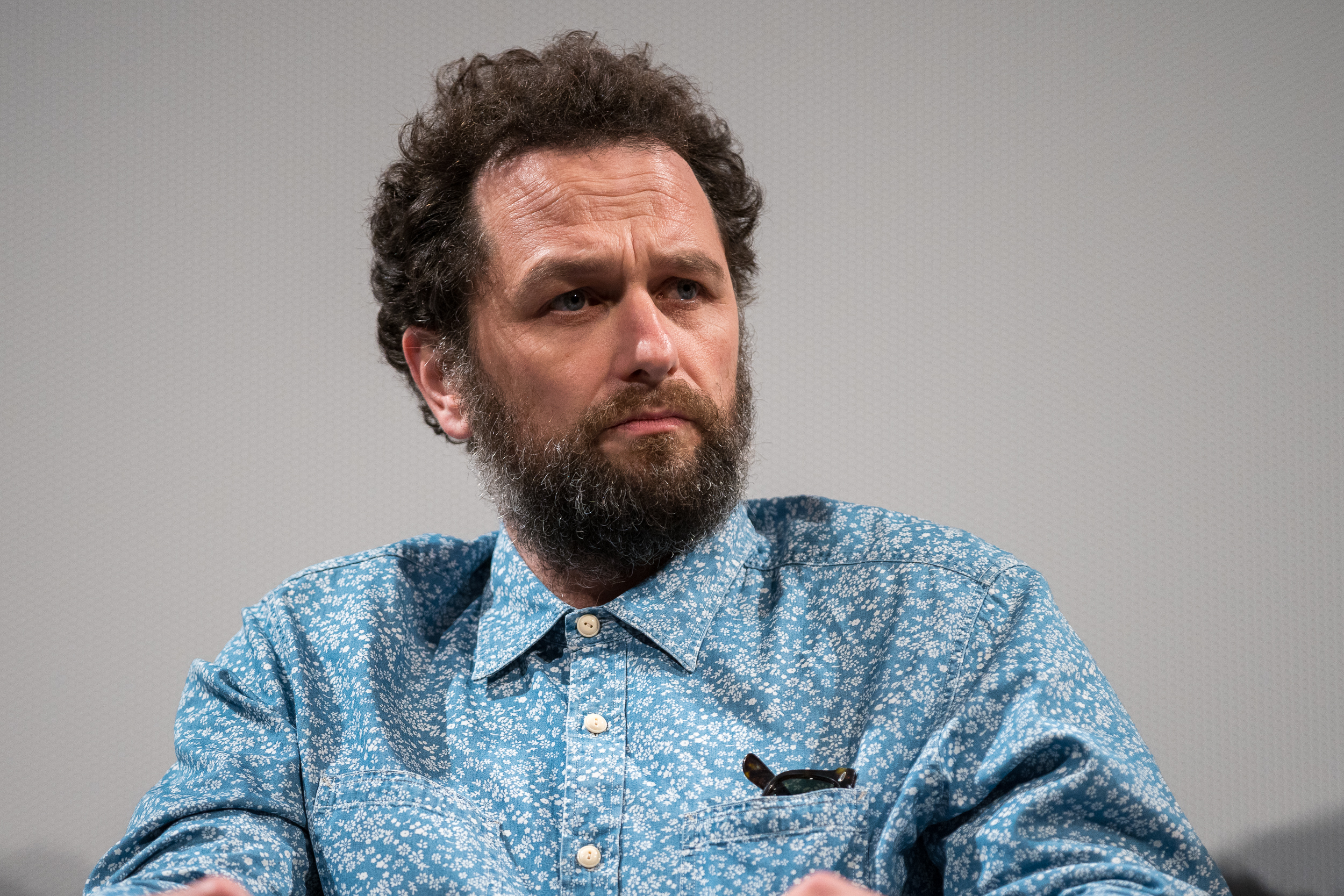The image features a man with short, curly, dark brown hair and possibly blue eyes, though the exact color is uncertain. He has a full beard and mustache that extend almost to his shirt collar, with noticeable gray and white highlights. The man appears somewhat unhappy or worried and is looking at something off-camera. He is dressed in a light blue, long-sleeve button-up shirt adorned with a fine floral or paisley pattern, with white buttons fastened all the way to the top. The shirt's breast pocket holds a pair of sunglasses, showing just enough to suggest a tortoise shell frame. The background consists of a gradient of light to darker gray shades, casting a shadow in the bottom right corner of the image. The photograph captures the man from the chest up, with the overall composition indicating he is the central focus of the image.